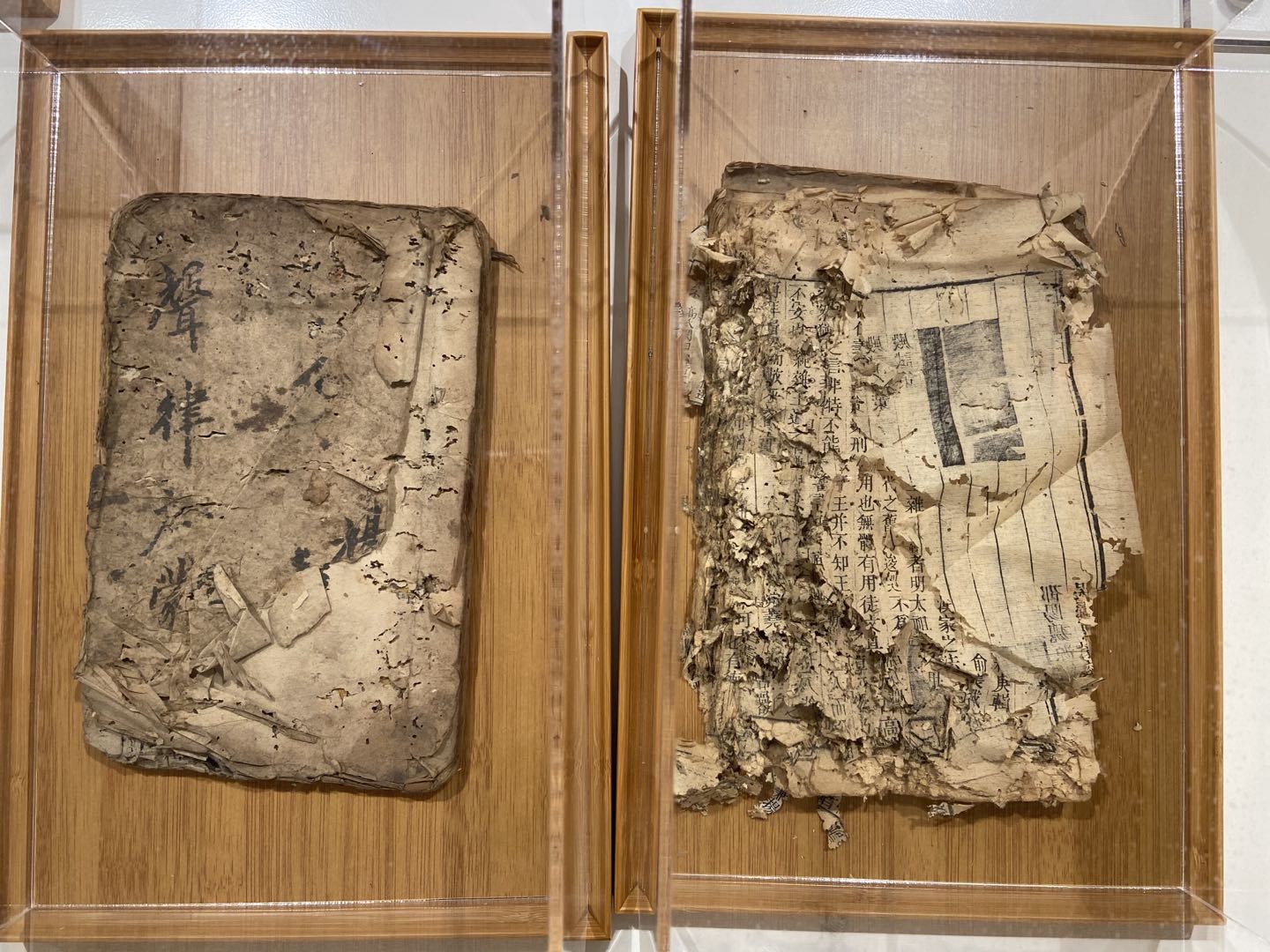This image depicts two meticulously preserved displays of ancient papers in a museum, presented side by side. On the left, a tablet-like arrangement features a group of overlapping papers, the topmost of which is significantly worn and tattered, exhibiting notable tears and missing sections. Clear Chinese characters are inscribed on this fragile sheet, offering a glimpse into the historical context of these documents.

To the right, a more deteriorated collection of papers is showcased. This stack is in far worse condition, with many sheets heavily torn and partially disintegrated. Despite their compromised state, the presence of additional Chinese writing is evident, extending the narrative of historical significance. Additionally, the upper right corner of one of these papers contains a faint image, although its details are obscured due to distance and decay.

Overall, these ancient documents are in a severely degraded condition, visibly worn from centuries of age and usage, yet they continue to hold invaluable insights into their era.